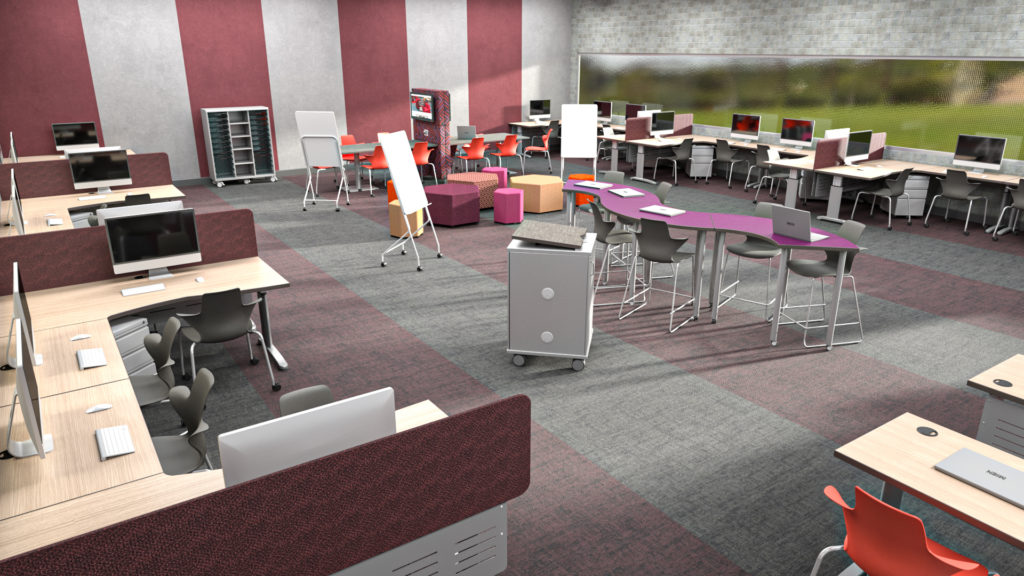The image showcases a spacious, open office area with a blend of functional workspaces and collaborative zones. The far wall features an eye-catching maroon and gray striped pattern, which complements the similarly striped carpet. Along the left side, there are shared cubicles arrayed as horseshoe-shaped desks, each equipped with four computer monitors. This configuration repeats on the far right side of the image, enhancing the symmetrical layout of the office. 

In the center, an array of tables with an assortment of seating options invites collaboration. One prominent table has a curvy, purple-topped design surrounded by tall chairs, doubling as a hub for group projects or team meetings. Several laptops are visible on the central tables, along with filing cabinets, shelves, and whiteboards, indicating a work-oriented environment. Additionally, a presentation chart and various colorful shapes that resemble seating pods or tables add to the functionality.

The back section houses multiple seats with computer screens and drawers underneath, highlighting the purposeful distribution of workstations. To the far right, a blurred window offers a hint of natural light. The color scheme of maroon, gray, and accent colors like purple and tangerine, coupled with white elements, weaves a vibrant yet cohesive aesthetic throughout the room.